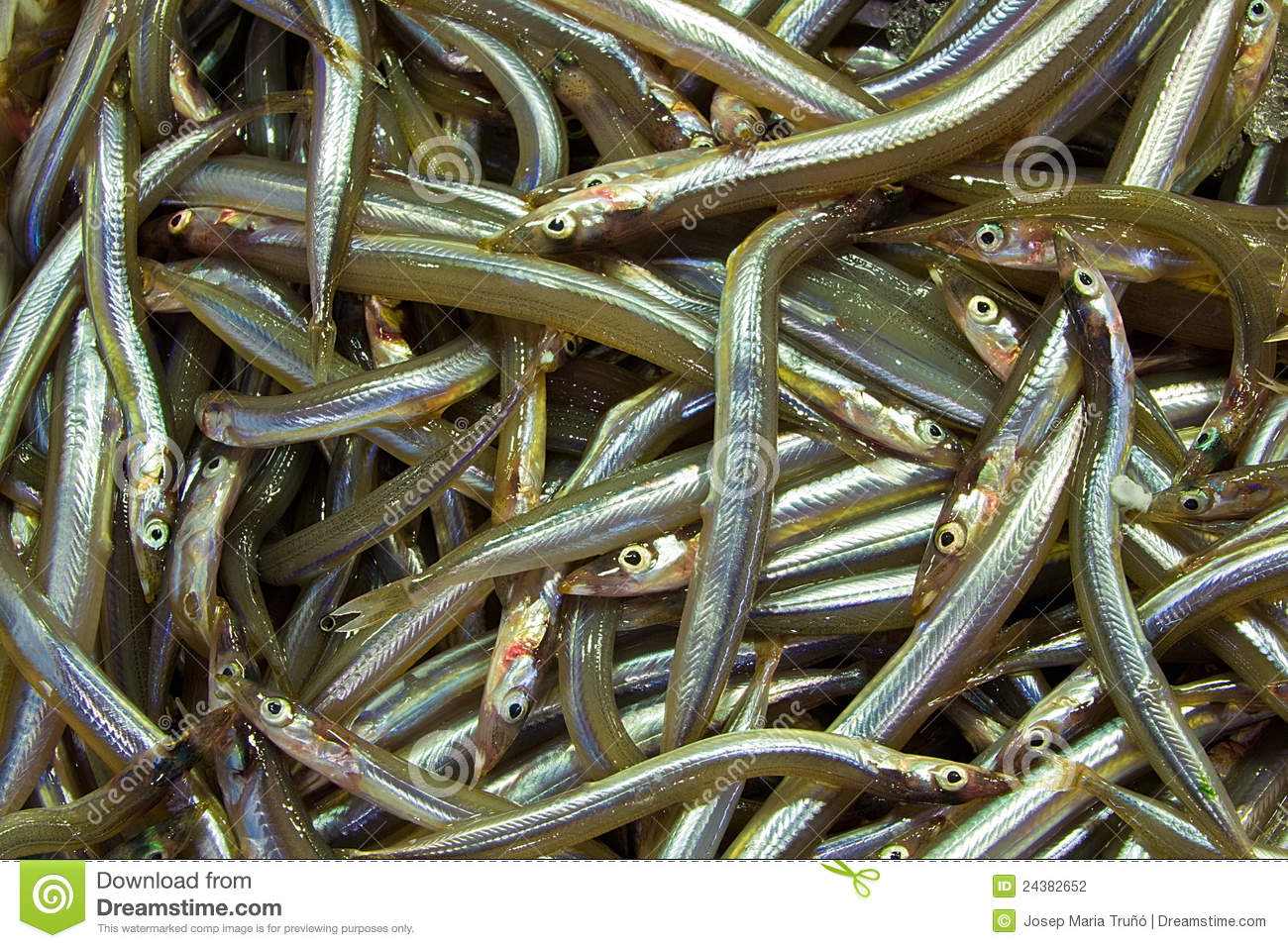In this detailed stock image from Dreamstime.com (ID 24382652) by Josep Maria Trujillo, we see a large pile of long, thin, silvery fish spread out in a dense heap. The fish exhibit a slight iridescence, particularly around the head, with subtle rainbow reflections highlighting their slick, slimy bodies. The sharp, pointed noses and small, distinctive eyes—black pupils set in off-white—add to their striking appearance. The photo's close-up perspective accentuates the sheer number of fish, stacking them in a visually overwhelming array with no significant variation other than their sizes, from smaller specimens to larger ones. Overlaying the image is a diamond checkerboard pattern and multiple swirl watermarks from Dreamstime, ensuring the image's secure stock status. At the bottom, a horizontal white bar contains crucial details: "Download from Dreamstime.com" marked on the left, green squares with ID number 24382652, and the photographer’s name, "Josep Maria Trujillo, Dreamstime.com," along with a distinctive green banner featuring a white swirl on the far left.